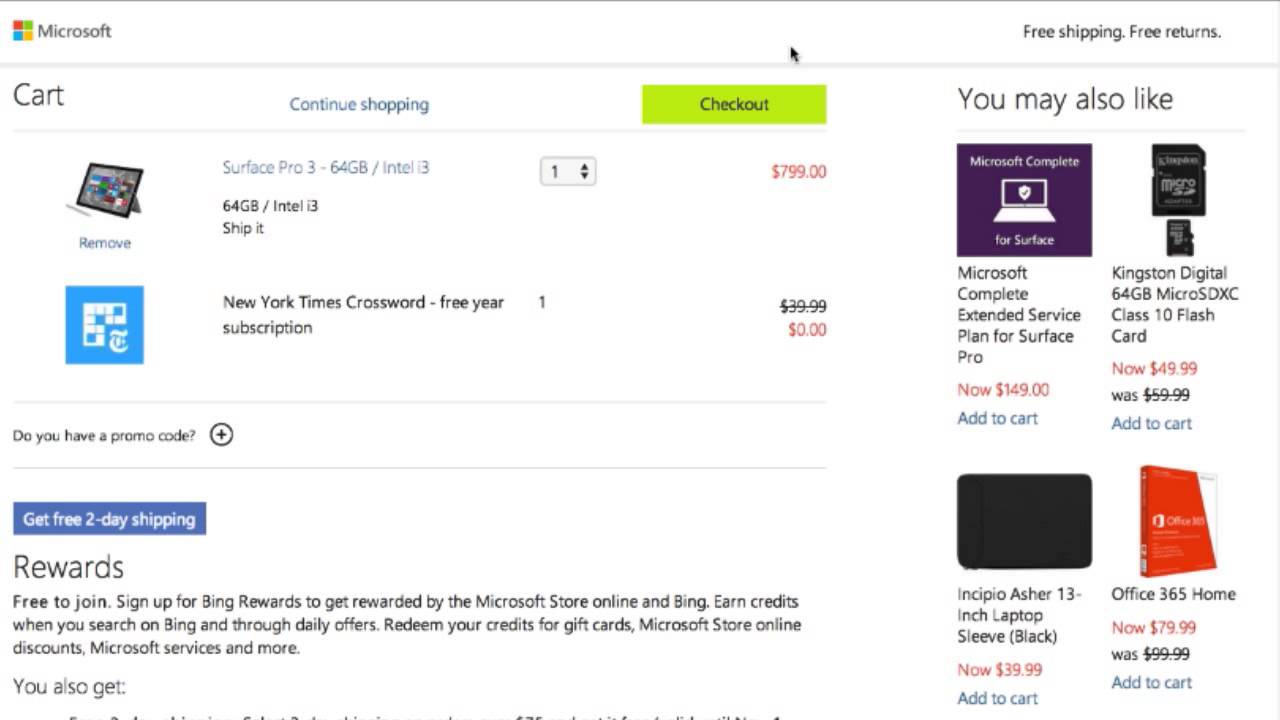The image depicts a Microsoft website featuring an active shopping cart. In the upper right corner, there's a prominent banner advertising "Free Shipping and Free Returns." Below this, the shopping cart section offers two action buttons: a grey "Continue Shopping" button and a green "Checkout" button. The cart currently contains two items: a "Microsoft Surface Pro 3 64GB Intel Tablet" priced at $799 and a subscription for the "New York Times Crossword (one year)" listed as free, costing $0.

Beneath the cart summary, there’s a promotional banner that reads, "Get 2-day free shipping with rewards" and notes that joining is free. This offer includes a brief description emphasizing the benefits of the rewards program.

Occupying about one-third of the right side of the screen is a suggestion panel titled "You May Also Like." It features four recommended products: a "Microsoft Complete Extended Service Plan for Surface Pro," a "Kingston Digital 64GB Micro SDXC Flash Card," an "Incipio Asher 13-inch Laptop Sleeve," and an "Office 365 Home Edition" subscription. Each of these items is accompanied by an "Add to Cart" button.